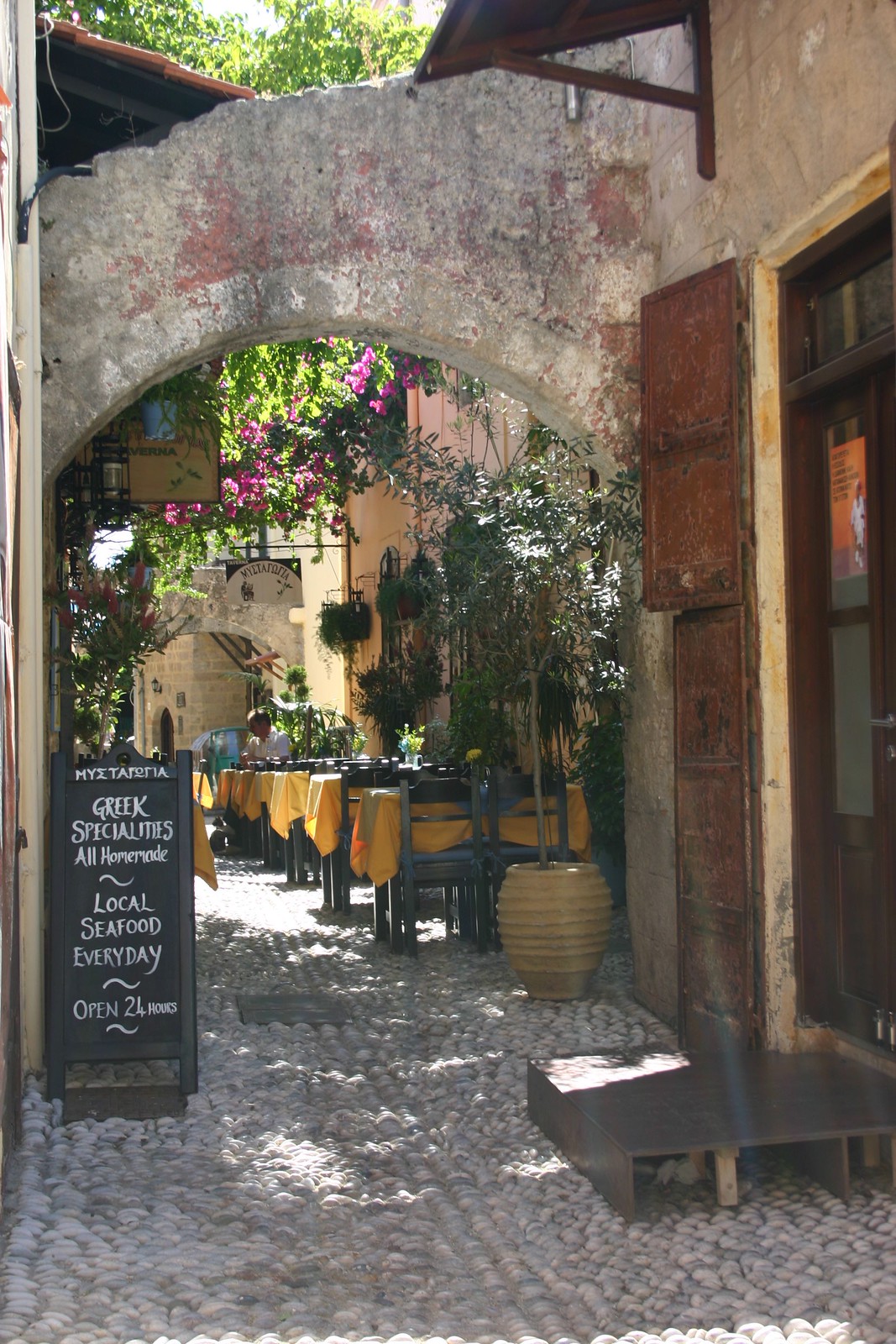The image depicts a charming, open-air cafe nestled within a pedestrian passageway that exudes an old European allure. A prominent black chalkboard sign with white writing on the bottom left advertises "Greek Specialties, all homemade, local seafood every day, open 24 hours," clearly signaling the cafe's offerings. The street paved with rough, vintage cobblestones leads towards a stone archway, under which the cafe's seating area is situated. All the tables, adorned with vivid yellow tablecloths and paired with dark wood or black chairs, are arranged towards the right side of the passageway. The facade includes a rustic brown doorway with shutters and a step on the far right. Ivy and flowering vines cascade along the walls, complemented by greenery from large pots and hanging flower baskets. Suspended wrought iron signs add to the picturesque atmosphere. A man is seen sitting at one of the tables in the backdrop, under dappled daylight filtering through the space, hinting at a tranquil daytime setting in this semi-shaded, inviting locale.